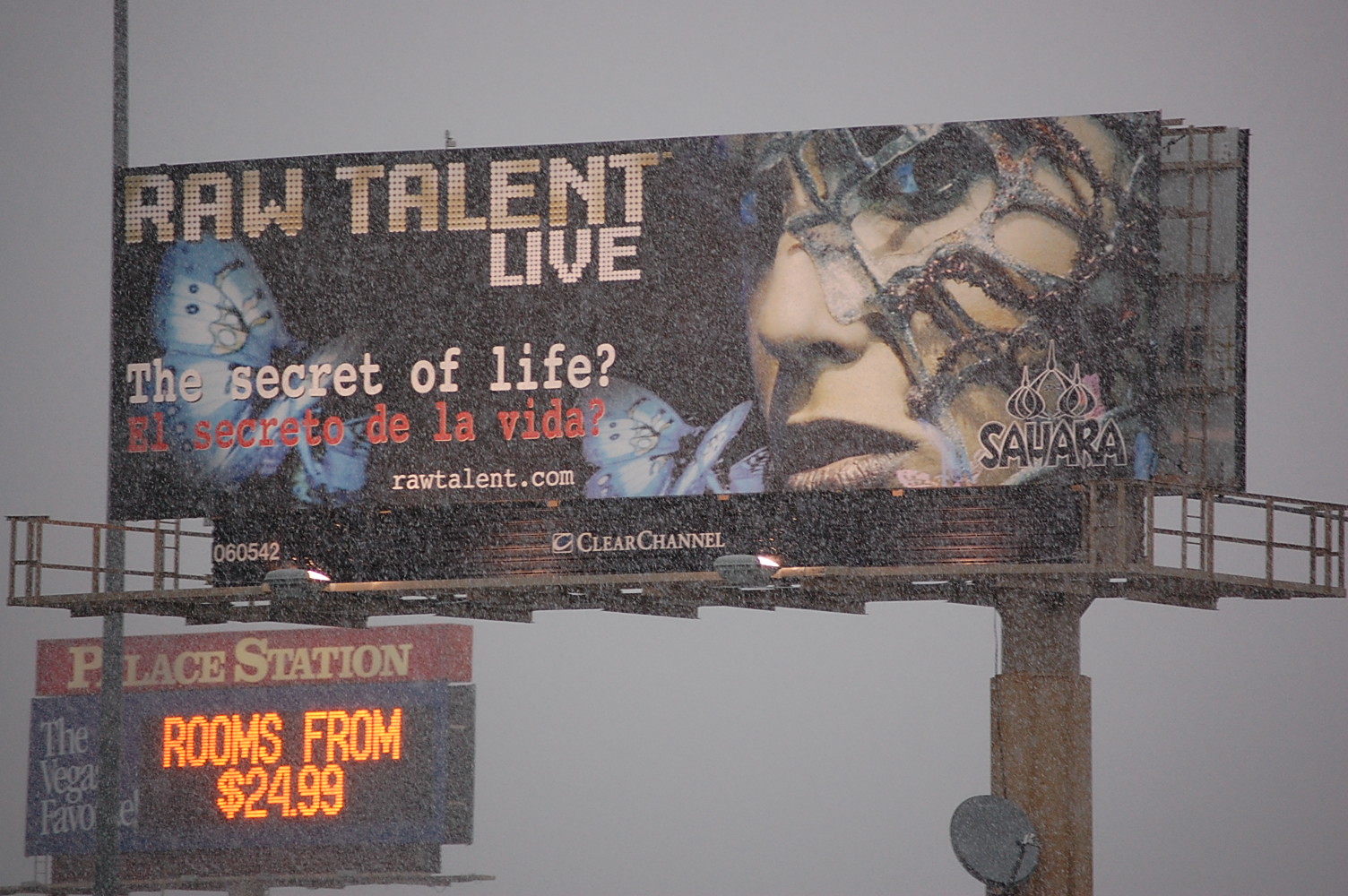This photograph showcases two prominent billboards set against the urban landscape. The first, an imposing structure mounted on a brown metal platform, features a striking advertisement with a black background. Dominating the visual is the face of a woman draped in a brown net-like material, her lips accentuated with bold, black lipstick. Emblazoned in gold letters, the billboard declares "Raw Talent Live," while the white font underneath reads "Secret of Life," accompanied by its Spanish translation "El Secreto de la Vida" in red font. The woman’s face is overlaid with the name "Sahara" in black font. Additionally, the website "RawTalent.com" is displayed in white font.

Beneath this vivid advertisement is a second billboard with a distinctive red top. In white font, it promotes "Palace Station" and proudly proclaims "The Vegas Favorite" on one side. Integrated into this display is a digital section that announces "Orange Rooms from $24.99," offering a glimpse into the accommodation deals available at the establishment.